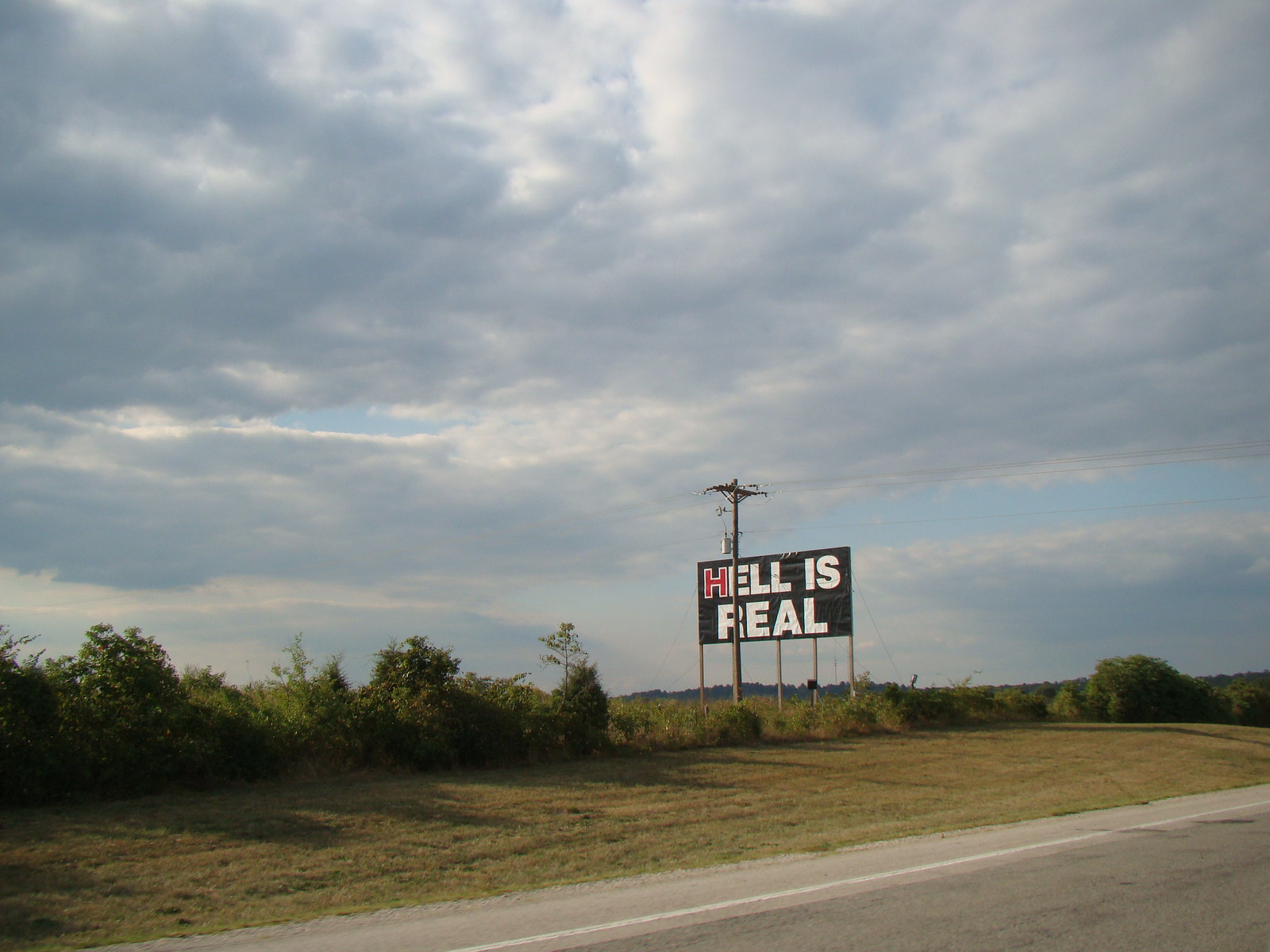This outdoor photograph captures a scene on a gray stone roadway, flanked by patches of green and light green grass on either side. The road's edge is marked by a white line. On the left side of the frame, and continuing along both sides, various green shrubs and trees of differing heights can be seen. Dominating the middle ground is a large, rectangular black sign with the bold white message "HELL IS REAL," except for the "H," which is strikingly red. This sign is supported by five wooden posts. Positioned in front of the sign is a tall wooden telephone pole with horizontal wires extending outwards. Above, the sky is mostly cloudy, featuring a mix of gray and fluffy white clouds, with occasional glimpses of blue sky peeking through.